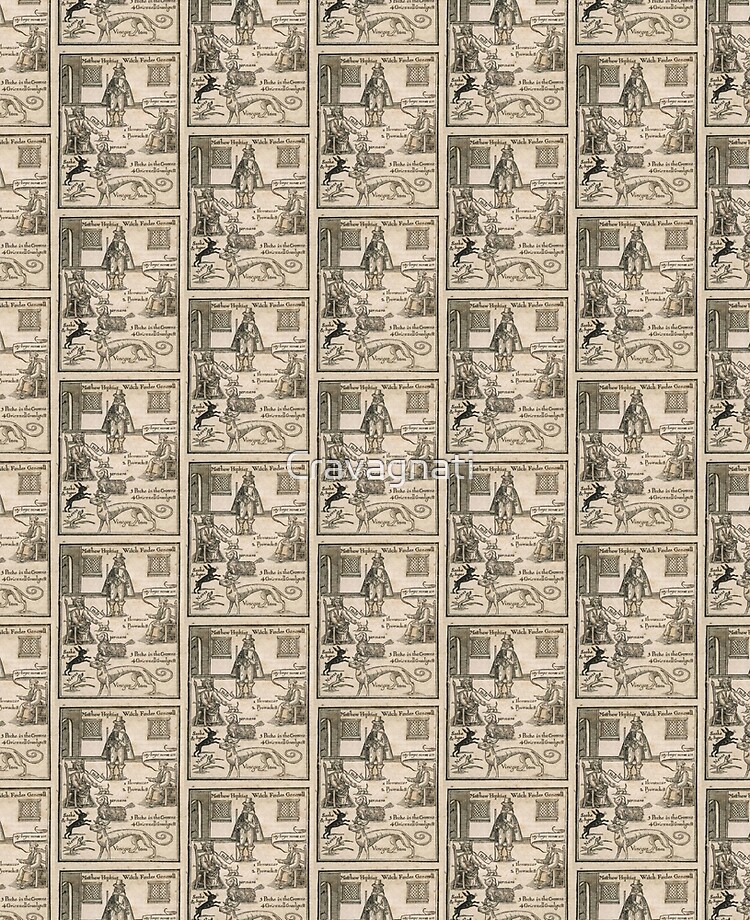This vertically-rectangular image features a repeated cartoon strip rendered in black and sepia tones, giving it a vintage feel. The image is divided into five full vertical strips of the cartoon, with partial strips visible on the extreme left and right edges. Separating each strip are staggered, brownish-colored lines that offset each strip halfway, adding a visually interesting layering effect. There is no visible border framing the image. Centrally located in the image is the word "Navagnata" written in white letters, accompanied by a circle figure that resembles a copyright symbol, heightening its distinctive and artistic appearance.